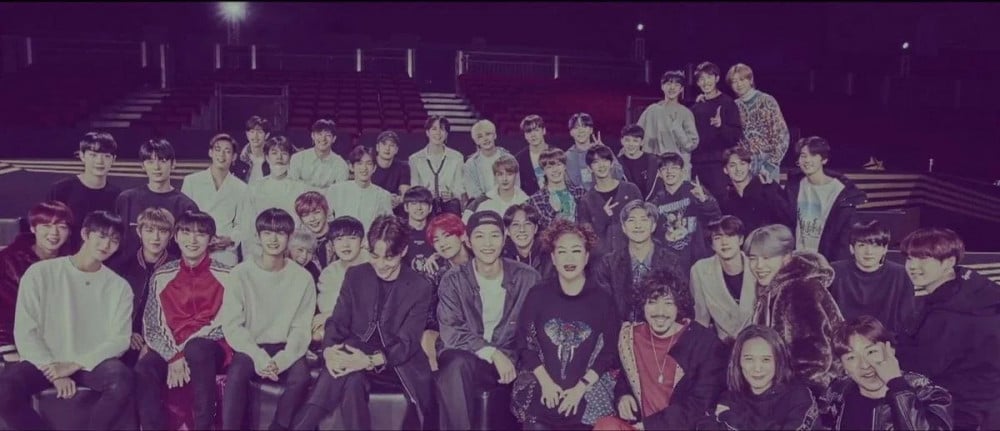The photograph depicts a large group of mainly East Asian teenagers in an auditorium or theater with a blue filter effect. The group consists of at least four rows of well-groomed young people, some standing and others sitting, all appearing very happy and engaged, many of them smiling and flashing peace signs. The majority are dressed in long-sleeved t-shirts, jackets, or sweatshirts. Notably, most have dark hair, though a few individuals have dyed hair—either red or blonde. At the center of the front row, a woman with short brown curly hair wearing a black long-sleeved T-shirt with an elephant logo on the chest stands out. In the background, the auditorium's elevated spectator area is visible, filled with many rows of empty red chairs, emphasizing that the attention is focused on the group in the foreground.